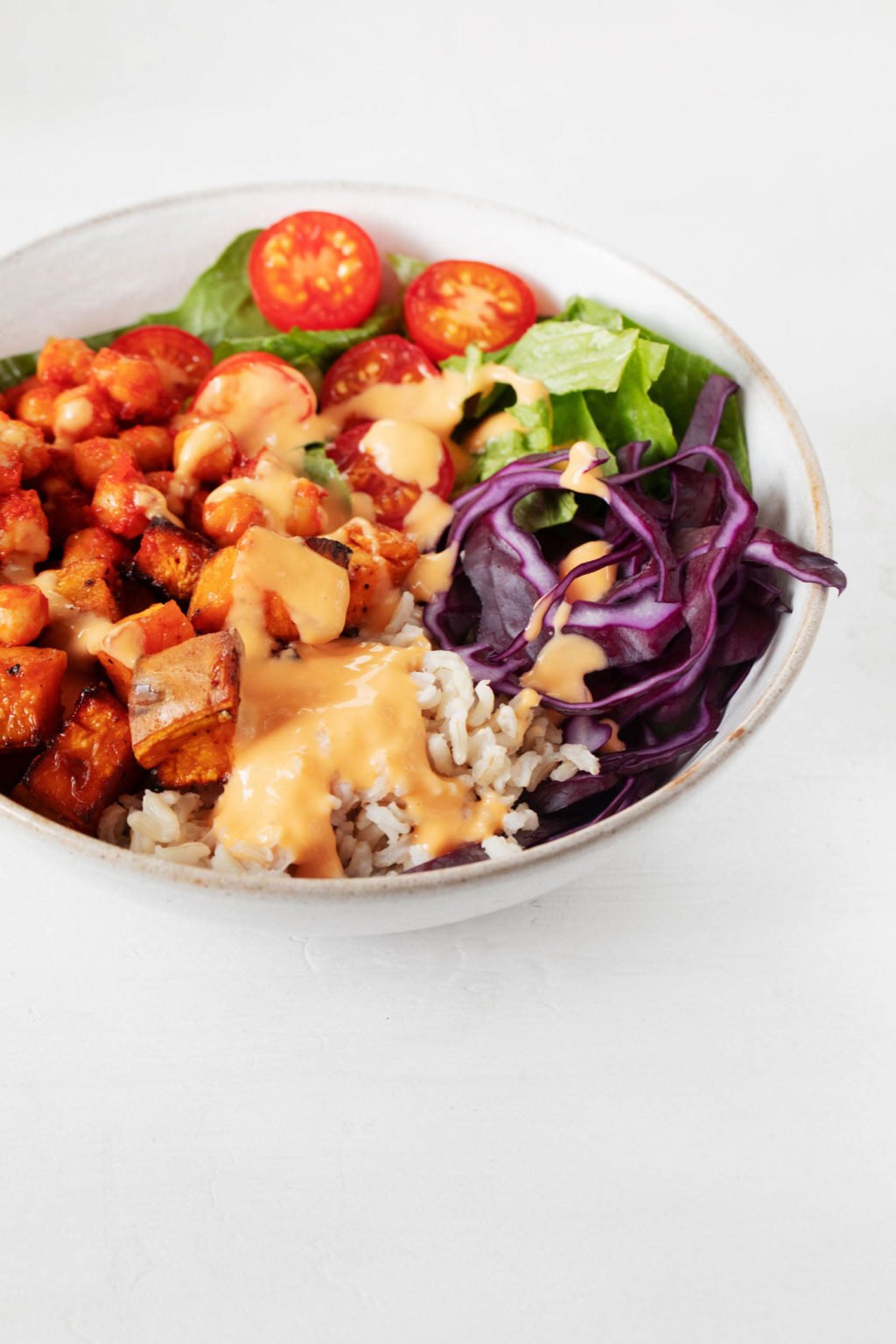This detailed photograph showcases a vibrant and healthy salad arranged in a large, white bowl against a light grey backdrop. The various ingredients are meticulously separated rather than tossed. On the left side of the bowl, there is glazed chicken, adding a savory element with its appealing red tinge. Scattered among green lettuce leaves are cherry tomatoes sliced in half and dressed with a light orange Thousand Island dressing. The right side features finely sliced purple cabbage. At the bottom, a base of brown rice or quinoa is visible, also dressed in the same light red or Thousand Island-like sauce. Amidst these main components, there appear to be some white beans and additional pieces of chicken. The entire presentation emphasizes a wholesome, nutritious meal with a delightful mix of colors and textures, capturing the essence of a fresh and appetizing salad.